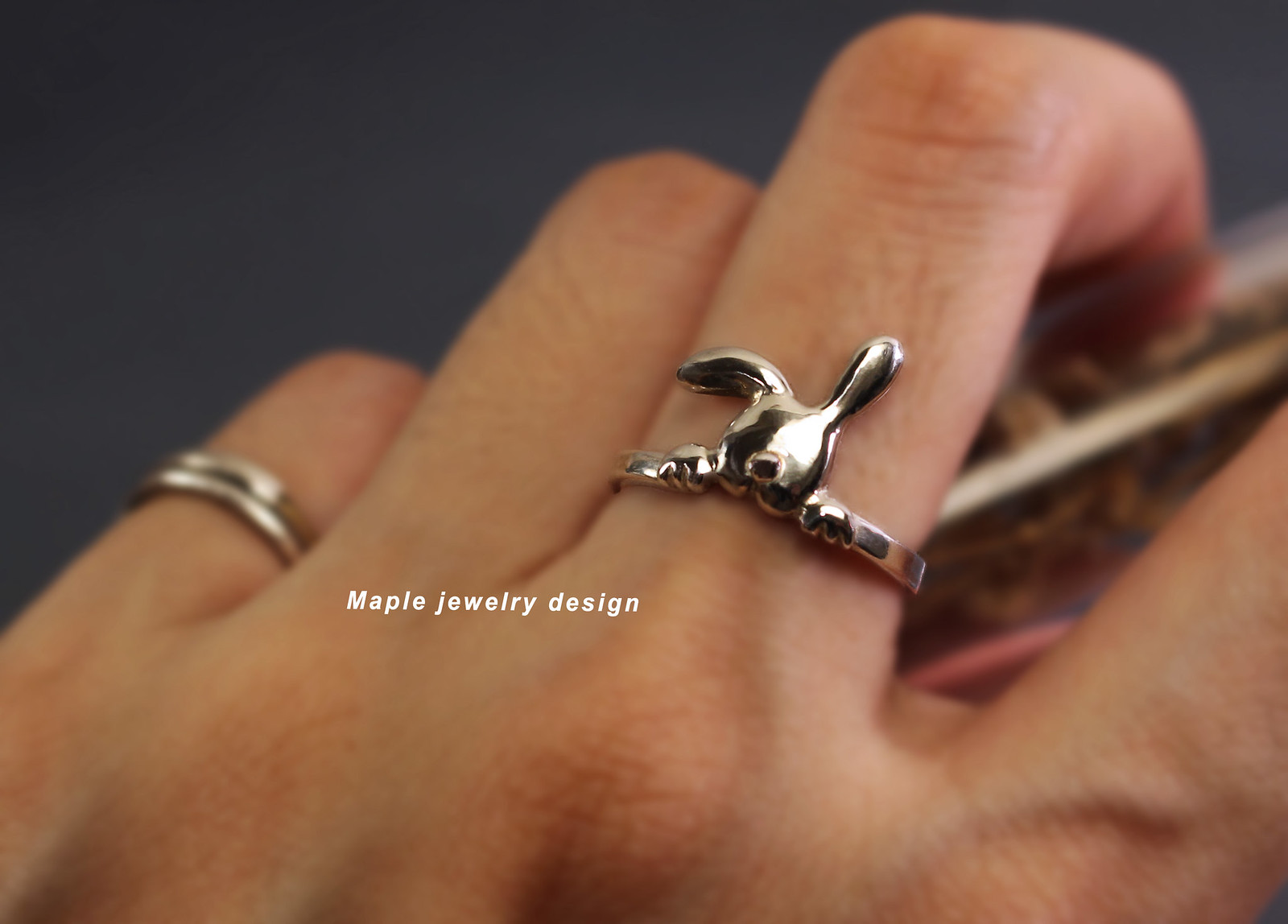The image showcases an extreme close-up of a Caucasian person's hand, specifically focusing on their middle finger adorned with a striking piece of custom jewelry. The ring, made of shiny silver metal, features a distinctive design of an animal's head, which resembles a bunny. The bunny's head occupies the center of the ring; one ear stands upright while the other flops halfway sideways, adding a unique, whimsical touch. The bunny's little hands clasp both edges of the ring band, and its nose is slightly square-shaped. Additionally, the person also has a simple metal band on their pinky finger. The background of the image is a deep navy blue, and subtle veins are visible on the person's fingers. Accompanying the close-up shot, small white text reads "Maple Jewelry Design," emphasizing the creator of the intriguing ring.